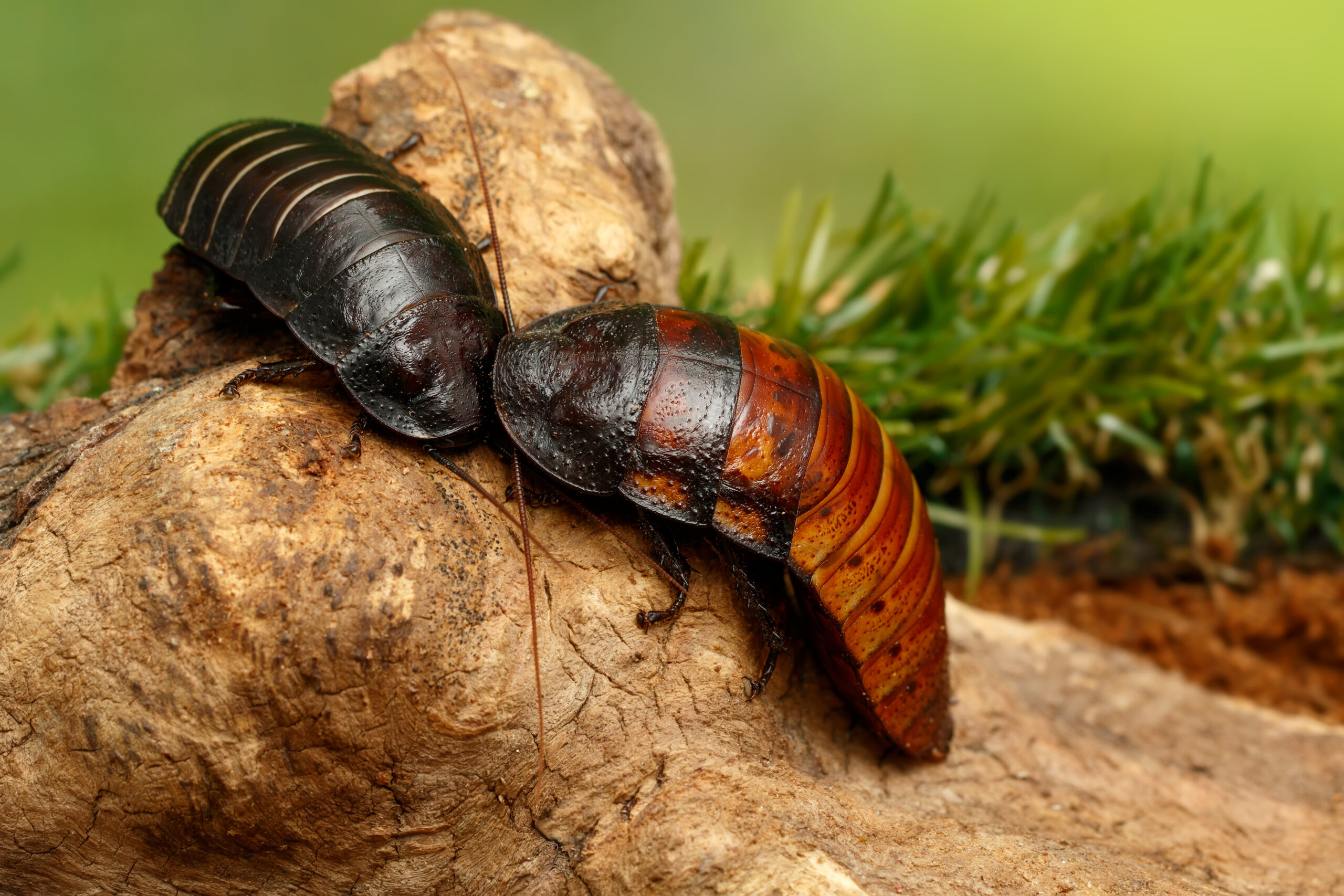The image depicts two large cockroaches situated on a piece of wood, which stretches across the entire frame from left to right, then narrows down towards the bottom right. The wood serves as a platform against a green background with visible grass or weeds. The photograph is taken at a slight angle from the front and above, giving a detailed view of the insects. The cockroach on the left is entirely black, shiny, and appears to have indentations on its back, with its head facing the camera and its tail toward the top of the page. The cockroach on the right, slightly larger and brown with black speckles, has a shiny shell with distinct indentations and stripes. Its head touches the black cockroach, facing left while its tail is angled downward. Thin brown antennae are visible on both cockroaches, adding to the detailed and textured appearance of these likely African species.